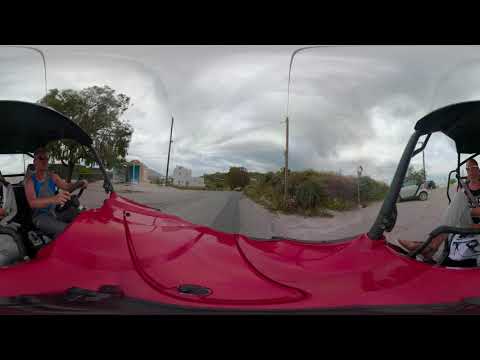This color photograph, taken in landscape orientation, has the appearance of a panoramic image created by combining three separate photographs. A black horizontal stripe spans across the top and bottom borders of the image. At the left side, a red vehicle, resembling a golf cart or dune buggy, is depicted with its driver wearing a blue shirt, dark pants, and sunglasses. In the center, the scene looks down a gray road flanked by grass, trees, and bushes, leading towards a two-story light cream or beige house. On the right side of the composite image, we see the passenger of the red vehicle, wearing a white shirt with black designs and dark pants, and white sunglasses. The vehicle has a black roof with connecting black bars. A silver smart car with black trim is visible in the background, parked by the roadside. This outdoor setting is under a blue sky with white feathery clouds, capturing a moment that blends the street-side activity with the greenery and structures around.